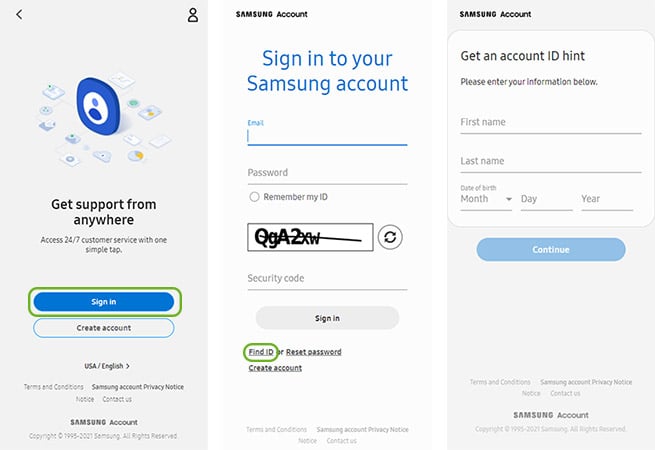The image showcases three consecutive mobile screenshots, each visually organized to demonstrate a different phase of user interaction with a service platform.

**Screenshot 1:**
- **Header Text:** "Get support from anywhere"
  - Positioned above an illustrative icon featuring multiple devices including a camera, tablet, phone, and gaming controller, emphasizing ubiquitous support.
- **Background:** Dark grey to black gradient, creating a sleek and modern look.
- **Main Text:** "Access 24/7 customer service with one simple tap."
- **Buttons:**
  - "Sign In" (Blue button)
  - "Create Account" (Green rectangle outlining the blue "Sign In" button)

**Screenshot 2:**
- **Title:** "Sign in to your Samsung account"
- **Form Fields:**
  - Two input boxes for "Email" and "Password".
- **Options:**
  - A checkbox labeled "Remember my ID".
- **Security Verification:**
  - A CAPTCHA code input field.
- **Action Buttons:**
  - "Sign In" button.
  - "Find ID" (Text circled in green for emphasis)

**Screenshot 3:**
- **Title:** "Samsung account"
- **Subtitle:** "Get an Account ID hint"
- **Form Instruction:** "Please enter your information below."
- **Form Fields:**
  - Input boxes for "First Name", "Last Name", and "Date of Birth".
- **Button:** "Continue" (Blue button)

Each screenshot methodically guides the user through the process of accessing support, signing in, and creating an account, with clear instructions and visually distinct action buttons.